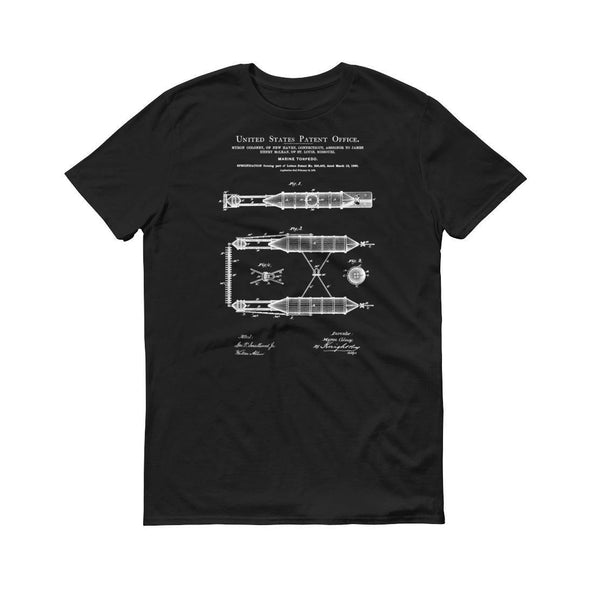This is a photograph of a black, short-sleeved t-shirt laid out on a solid white background. The t-shirt features intricate white text and drawings on the front. At the top, it reads "United States Patent Office" in crisp white letters. Below the title, the text becomes blurry and illegible. Beneath the text, there are several detailed diagrams that appear to represent a historical marine torpedo, reminiscent of early submarine torpedoes. The top diagram showcases a longer cylindrical shape, while two shorter diagrams are positioned below it, connected by an 'X' and a distance measuring bar. Additional lines of blurry text are situated beneath the diagrams. The t-shirt does not have a visible tag, and only the front side is shown in the photograph, making it ideal for display or sale on a website.